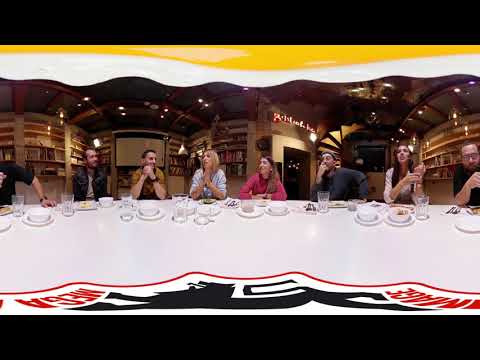The image is a small, horizontal rectangular photograph bordered by thick black bands at the top and bottom. It features a group of casually dressed people seated around a long, curved dining table covered with a white tablecloth. Approximately seven to eight individuals are visible, engaged in conversation, with white plates, bowls, glasses, cups, and saucers set in front of them, though the specific types of food are not discernible. The table, which spans the width of the photo, has a partial logo or emblem that is hard to read, appearing to be black and red, possibly spelling "mega." The background consists of tan walls, shelves, and doors, with some parts of a brown ceiling and illuminated lights suggesting a restaurant setting. A scalloped, white area above the photograph gives way to a yellow curved banner at the top edge of the image, enhancing the visual complexity. Overall, the scene appears to capture a moment of anticipation before dinner in a warm, casual atmosphere.